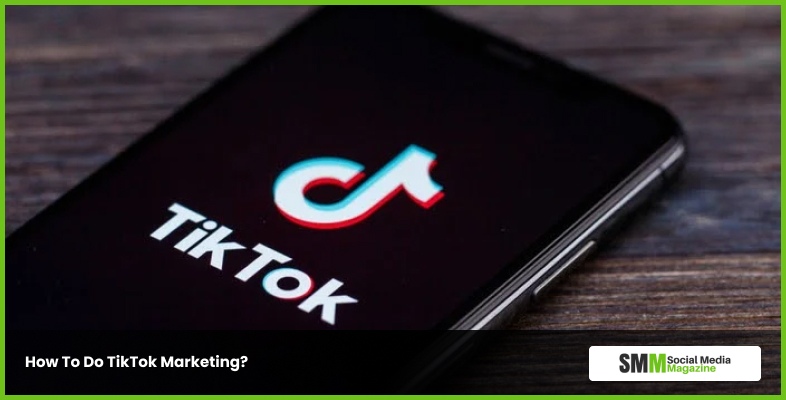A landscape-oriented screenshot from a tablet or desktop setup is framed with a distinctive lime green border. The backdrop within the image reveals a wooden surface, likely a table. Placed on this table is a black smartphone, positioned with its top half visible and screen angled toward the viewer. The phone displays the TikTok application, characterized by white letters with a rainbow outline and the iconic music note logo prominently occupying half of the screen.

On the right side of the phone, the volume buttons are visible, sleek and shiny. Below the TikTok display, text reads "How to do TikTok marketing?" in a white font set against a black box that spans the width of the screen's bottom. Adjacent to this text on the right, a white triangle features the acronym "SMM" for Social Media Magazine. The text within the triangle sports deep purple and lime green hues, indicative of the magazine's logo.